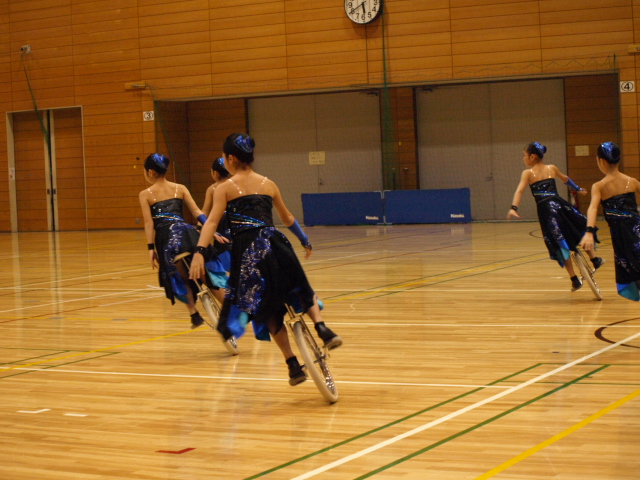The image captures a gymnasium setting with a white-brown wood-paneled floor that is highly polished and reflective, featuring multiple painted lines in shades of red, white, green, and yellow. In the background, there is a broad white-brown wood-paneled wall with two gray, garage-like rectangular doors. To the left of these doors is a set of smaller double doors. Mounted on the wall above the doors is a large black and white analog clock displaying the time as 5:40.

Five young girls with their backs to the camera are the central focus. They are performing or practicing a unicycle routine, riding unicycles with cream-colored wheels. Each girl is adorned in a strapless black dress, enhanced with blue highlights along the hem and waistline, as well as dark blue scrunchies holding their hair in tight buns. They are also wearing dark shoes, a blue arm warmer on their right arm, and a black wristband on their left wrist. The gymnasium, with its shiny floor and distinct markings, complements the coordinated and visually striking appearance of the girls performing in unison.